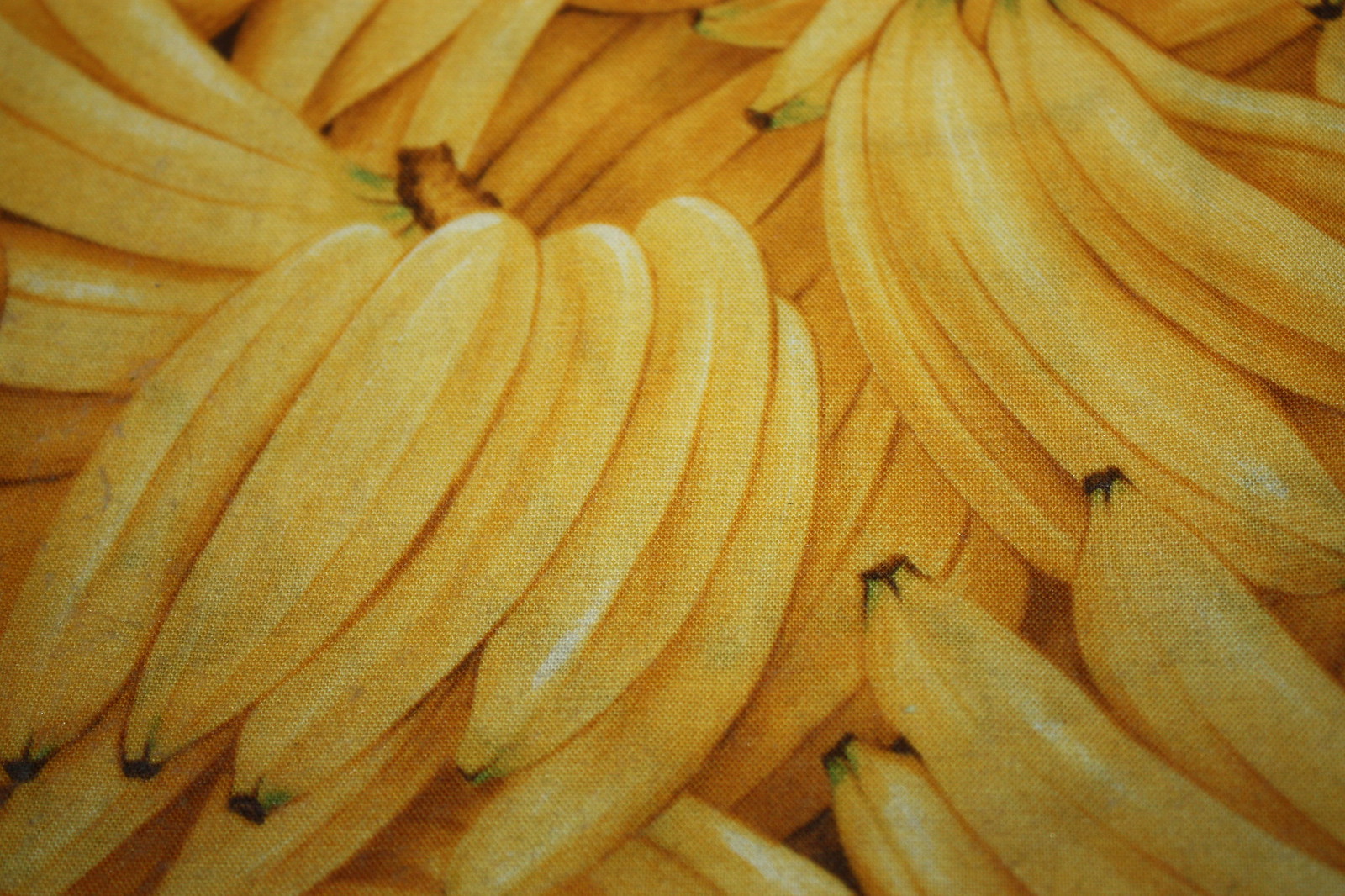This detailed, close-up image captures a realistic illustration of numerous vibrant, ripe bananas in various shades of golden yellow with faint hints of green and amber. Each banana bunch, consisting of five to seven bananas, displays brown-tipped stems and occasional green at the bottom, highlighting their freshness. Some bananas lie in neat clumps while others appear upside down or spread out, creating a layered, slightly chaotic arrangement with minimal gaps. Although set against a background of the same banana pattern, the woven fabric, possibly a cotton canvas, makes it difficult to discern the exact item it adorns. It could be a tablecloth, dish towel, or perhaps a tote bag, but the detailed artwork and reflective highlights give the impression of perfectly fresh bananas almost ready to be eaten.